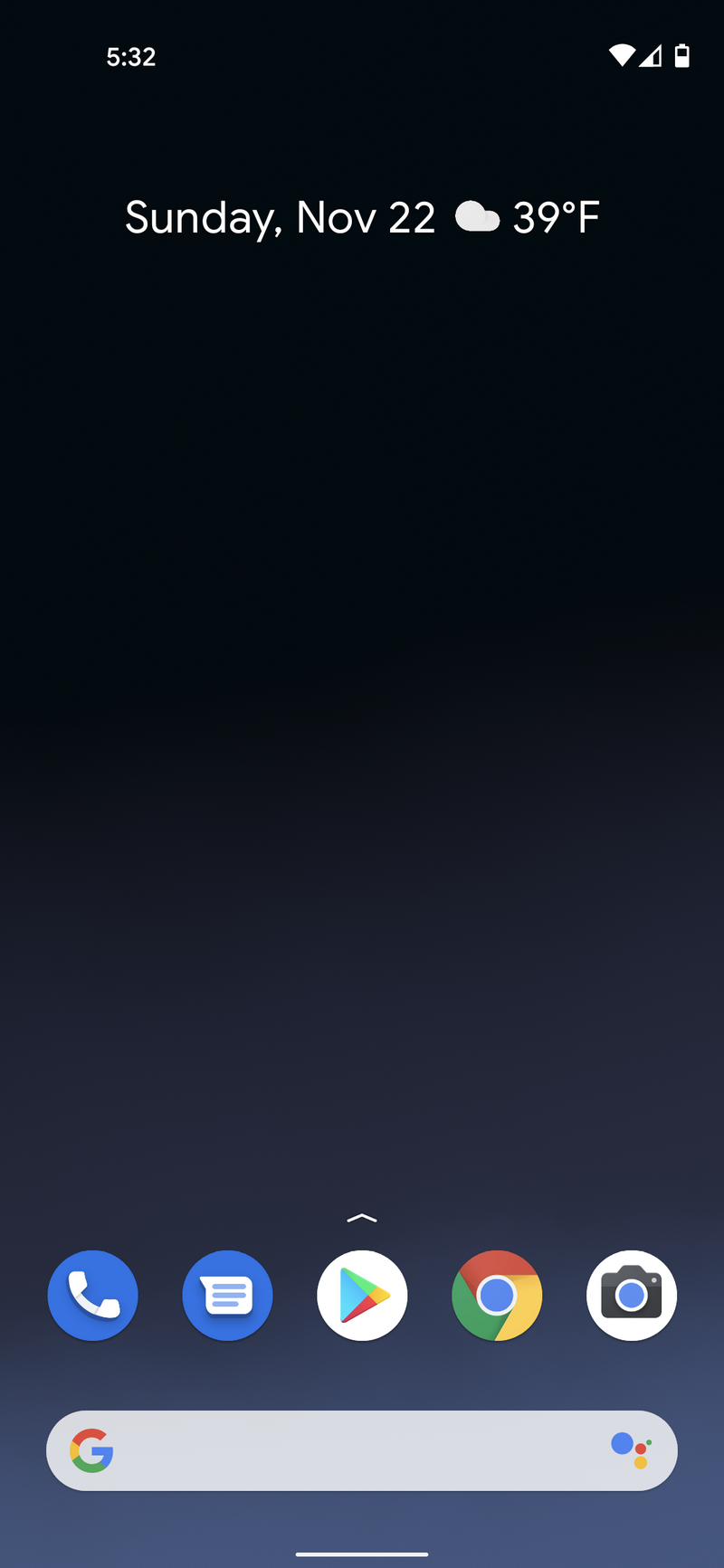This is a detailed description of a smartphone home screen screenshot. The background starts as a deep black at the top and transitions smoothly to dark blue and then to a lighter blue as you move down. At the very top, there's a timestamp reading "5:32," accompanied by a Wi-Fi signal icon and a battery icon showing approximately 50% charge.

Below these status icons, in white text, is the date "Sunday, November 22nd," and next to it, an icon of a cloud indicates the weather, displaying "39°F." 

The body of the screen is mostly clear with the fading gradient as the only design element. At the bottom of the screen are several app icons arranged from left to right: Phone, Documents, Google Play Store, Google (G) icon, and Camera.

Just above these icons, there's a search bar featuring the Google G logo in grey, with the right side displaying five dots in different colors: a large blue dot followed by smaller orange, red, lighter blue, and another Google G logo dot.